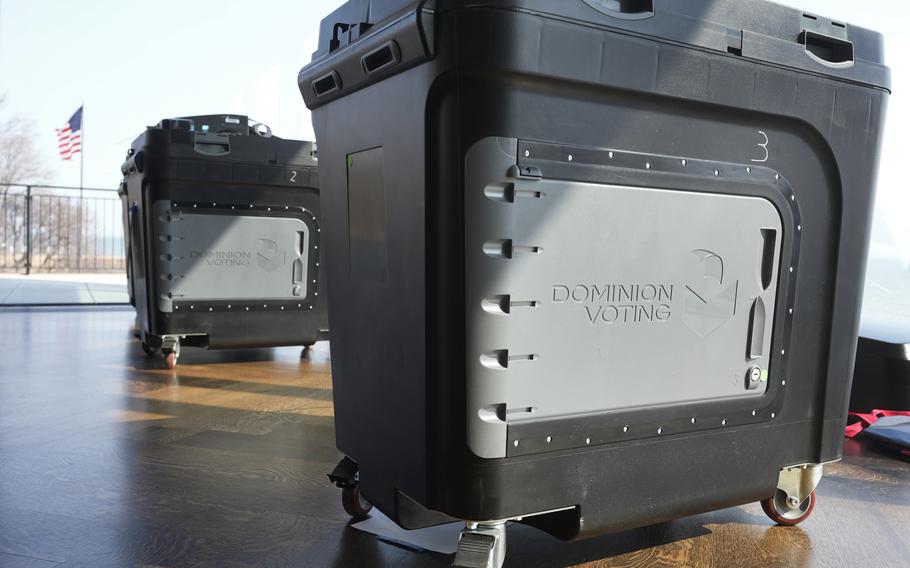This photograph depicts an outdoor setting with a clear, slightly hazy sky. Dominating the foreground are two large black and gray Dominion Voting boxes, each mounted on four silver metal wheels with red plastic trim. The boxes are centrally positioned, standing on what appears to be a brown hardwood floor. Each box features a gray locked door with a white number, three on one and two on the other, and a keyhole on the lower right side. Imprinted on the side of the boxes is "Dominion Voting," indicating their use in the voting process, likely for securely storing ballots. The background, out of focus to emphasize the boxes, includes an American flag on a pole to the left, adding a patriotic element. There's also black metal fencing and barren trees farther left, alongside a mix of wooden flooring and concrete sidewalk, all subtly lit by the sun, which enhances the outdoor ambiance.